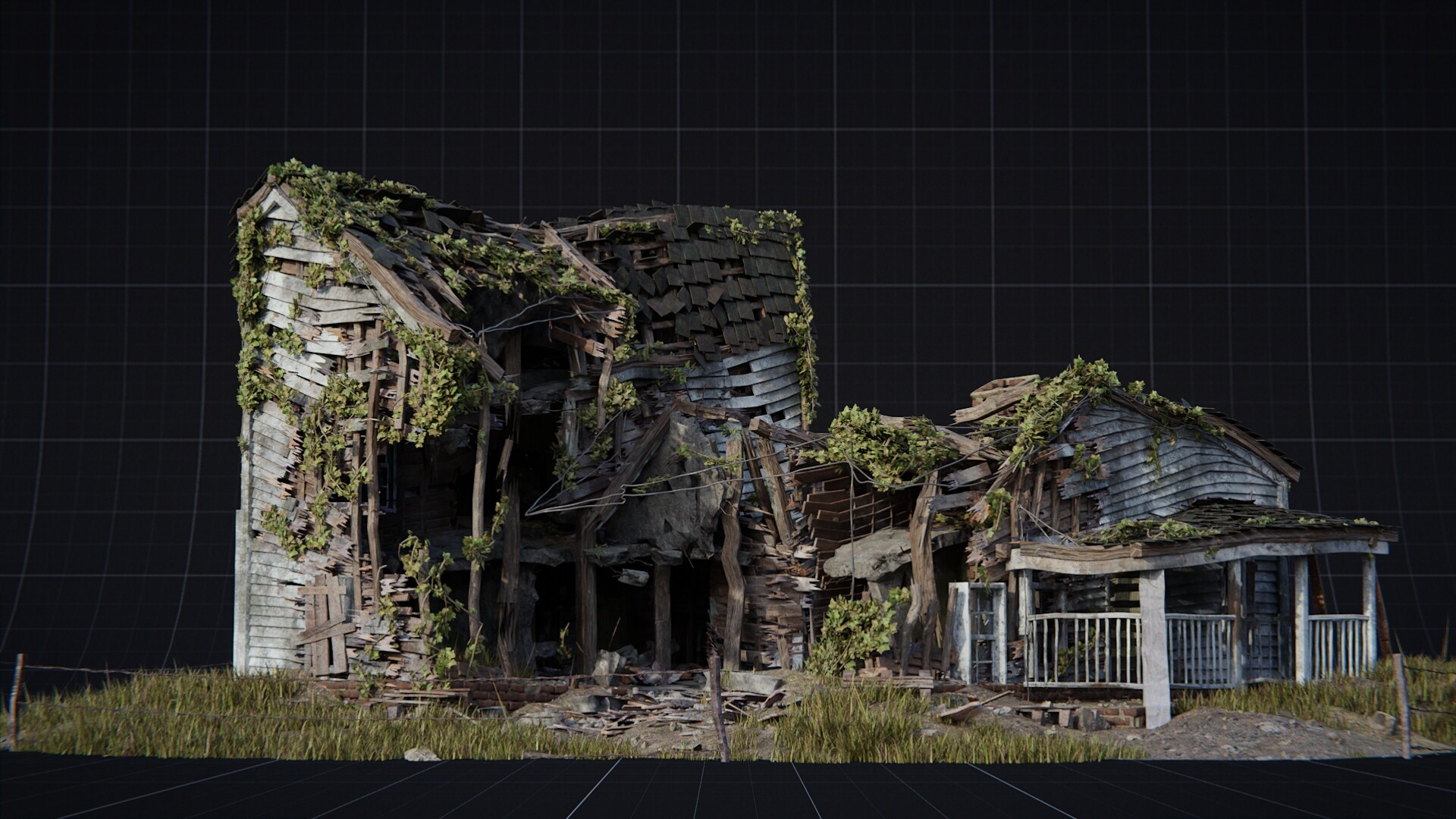The image depicts a computer-generated scene of two dilapidated wooden buildings against a black background, overlaid with a grid pattern of light gray horizontal and vertical lines. The taller building on the left appears to be a two-story structure. It is severely deteriorated with its front wall almost entirely missing, the roof caved in, and the wood rotten. Vines and plants have overgrown the structure, with some growing out from within the building itself. The smaller building on the right seems like an old house where the only parts still intact are the front porch railing and some column supports. The roof of this house is also sagging and compromised, with abundant plant overgrowth covering it. Debris and construction materials litter the foreground, with some grass visible among the detritus. A basic wire fence with wooden poles stands in front of the buildings, emphasizing the scene's overall neglect and ruin.